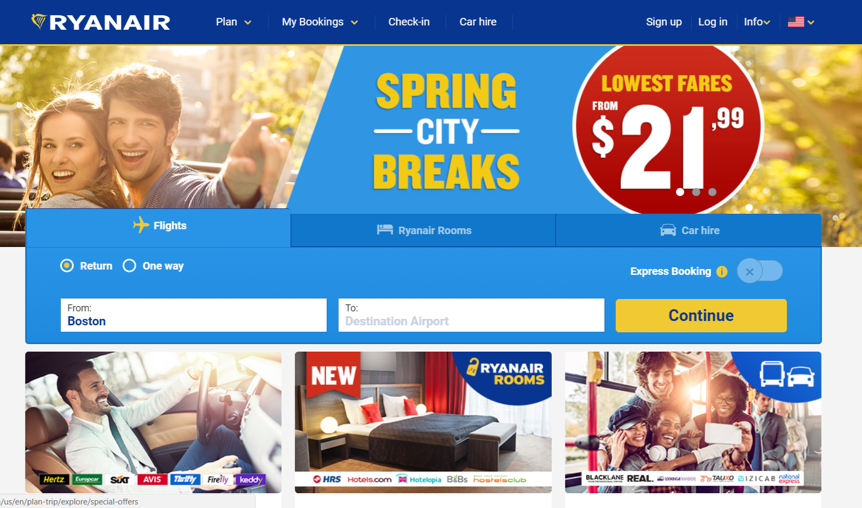The Ryanair website homepage features a prominent blue horizontal banner at the top, displaying the company's name, "Ryanair", alongside navigation options: "Plan", "My Bookings", "Check-in", "Car Hire", "Sign Up", "Log In", "Info", and a USA flag, likely indicating language or region preferences.

Below this banner, there is an image of a Caucasian couple promoting spring travel deals. To the right of the couple, the text reads "Spring City Breaks", with "Spring" and "Breaks" highlighted in yellow and "City" in white. Adjacent to this, a large circle advertises "Lowest Fares" in yellow, and "from $21.99" in white.

Further down, there are options for booking flights, Ryanair rooms, and car hire, each accompanied by relevant icons. The booking section offers choices between "Return" and "One Way" trips, with dropdown menus for selecting departure ("Boston") and destination cities, and a "Continue" button for proceeding with the booking. An icon for express booking is also present.

The page also features three promotional images. The first image shows a Caucasian man in a car, representing car rental services with logos from Hertz, Avis, Thrifty, and Enterprise. The middle image depicts a bed under the "Ryanair Rooms" section, on a blue background, featuring hotel partners such as Hotels.com. The final image shows a group of five happy people on a bus, promoting bus travel options. Each section provides a quick, visual guide to the various services offered by Ryanair, making navigation and booking straightforward for users.